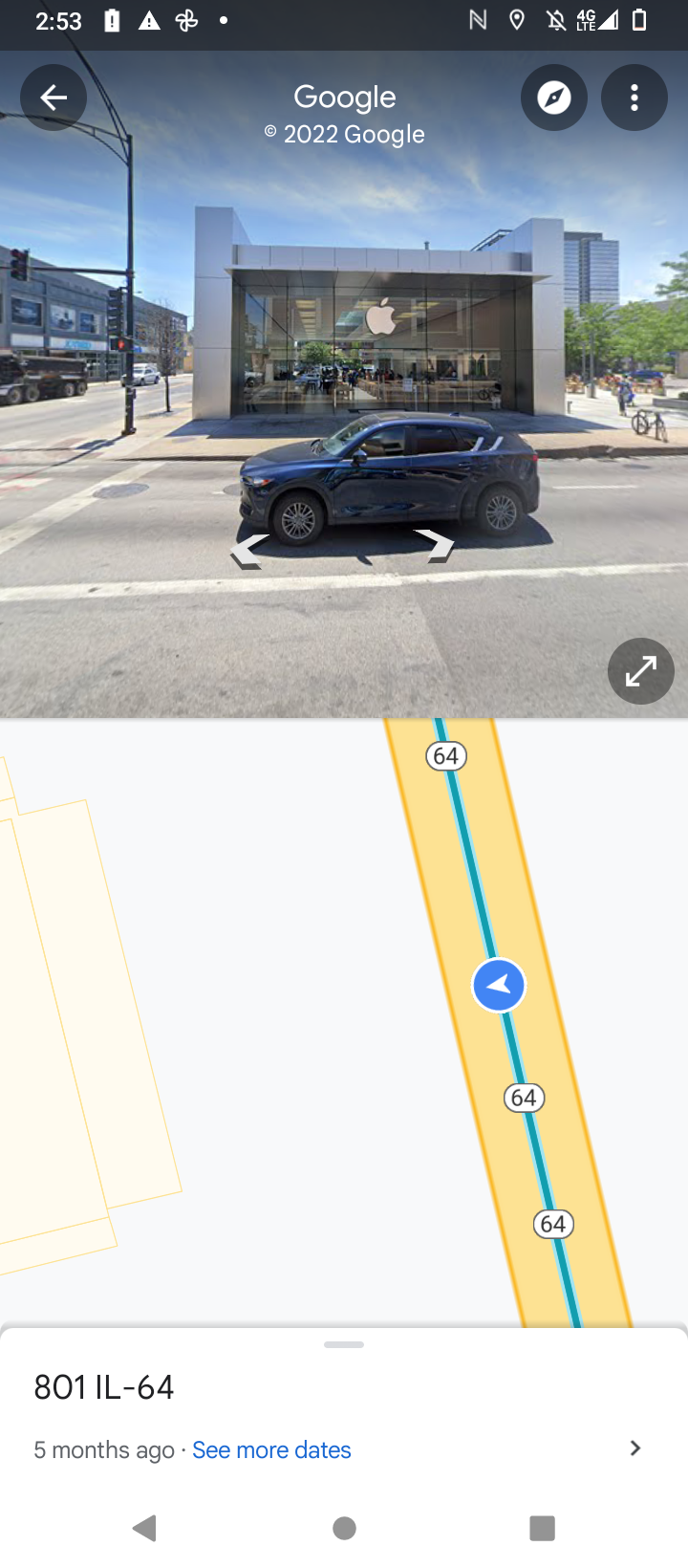The image appears to be a screen capture from a mobile phone of a Google Maps application, dated 2022. The primary focus of the image is a destination at the end of Route 54, which is displayed through a combination of map and road view elements. The destination seems to be an Apple store with a modern design, characterized by a white-framed exterior and large glass windows. In front of the store, there is a single parked car, which is gray in color, positioned on light gray asphalt. 

Additional on-screen details include map directions featuring a yellow road with a blue line in the center, labeled as Highway 64 (IL-64), which indicates the route. At the bottom left of the screen, there is text stating "A01 IL-64, five months ago," accompanied by blue text that says "see more dates." The upper left corner of the screen shows the time, 2:53, along with a fully charged battery icon and a warning triangle with an exclamation point. The screen capture evidently emphasizes a navigation route and features supplementary details, such as driving instructions, indicating a recent interaction with the Google Maps application.